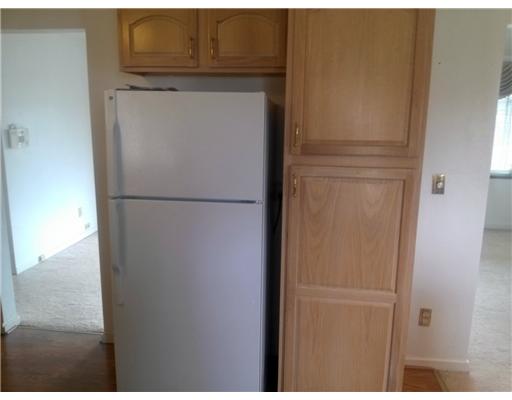The image depicts a portion of an empty kitchen within a house or apartment, focusing on a white refrigerator positioned against a light oak-colored cabinetry setup. The refrigerator, featuring a top freezer with a handle and a bottom refrigerator section with a handle, occupies a central spot in the frame. Above the refrigerator are two wooden cabinets with light gold handles. To the right of these, two larger cabinets stand from floor to ceiling, also adorned with light gold handles. The wall to the right of the fridge contains a light switch at the top and an electrical outlet at the bottom, with a window slightly further to the right that lets in daylight. The flooring in the kitchen appears to be brown linoleum. Through the doorway on the left, one can see into another room, presumably a living room, which has white walls, a white carpet, and a panel resembling a thermostat on the wall. A white column featuring gold-like fixtures is also visible from this angle. The overall scene captures a bright and vacant living space with simple, clean lines and a functional design.